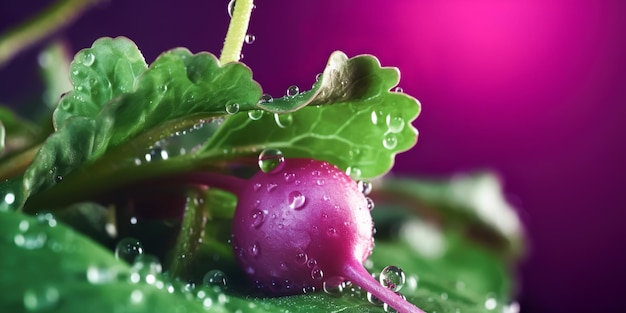This detailed, close-up photograph showcases a vibrant purple radish surrounded by lush green leaves, all adorned with water droplets that glisten like tiny bubbles. The radish, unusually purple throughout rather than the typical red and white, is centrally positioned in the image. A light from the right side casts a bright glare on its smooth surface, creating a distinct white spot. The background, an artistic blend of darker purple and fuchsia, provides a dynamic contrast, being darker in the upper left and lower right corners while brightening towards the upper right as if illuminated by a spotlight. The greenery, predominantly covering three-fourths of the image from the lower left towards the center right, features a mix of detailed and blurry leaves. The green stems and lobed edges of some leaves add textural variety, enhancing the overall freshness and vividness of the scene.